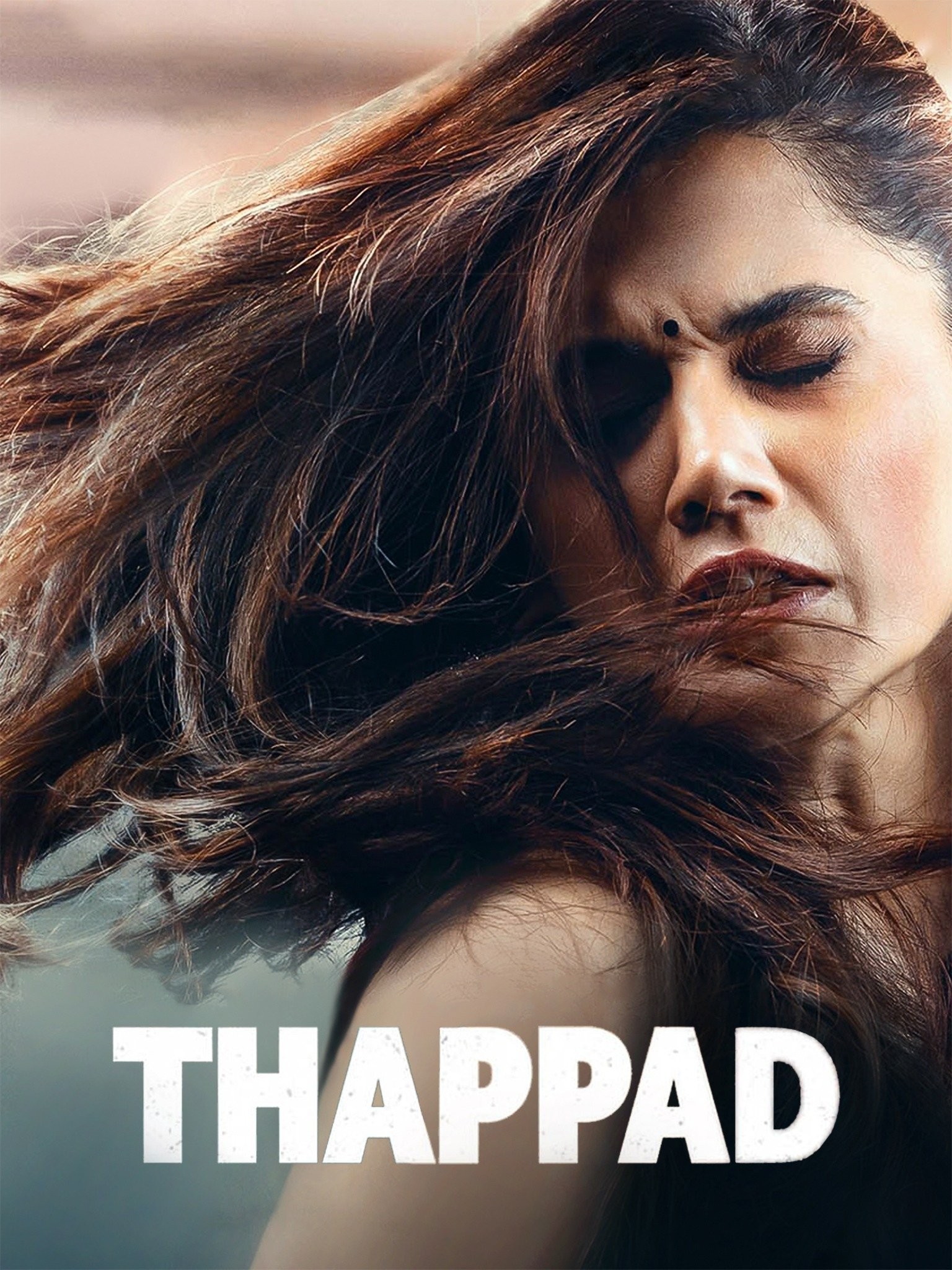The image depicts a likely South Asian woman with brownish-black hair cascading past her shoulders, visibly in distress. She appears to be grimacing and turning her head, causing her hair to flow dynamically to the left. Her eyes are closed, emphasizing the expression of pain or discomfort on her face. Distinctive features include a mole positioned between her eyebrows, brown eyeshadow, notable eyelashes with mascara, and maroon-colored lipstick. The woman is dressed in a sleeveless outfit, and her exposed arm is visible in the frame. The background transitions from a dark pinkish-red shade at the top to a light gray-blue tone at the bottom. Bold, white, uppercase letters spelling “THAPPAD” are prominently displayed across the image, likely indicating a foreign term, possibly the title of a movie or book.